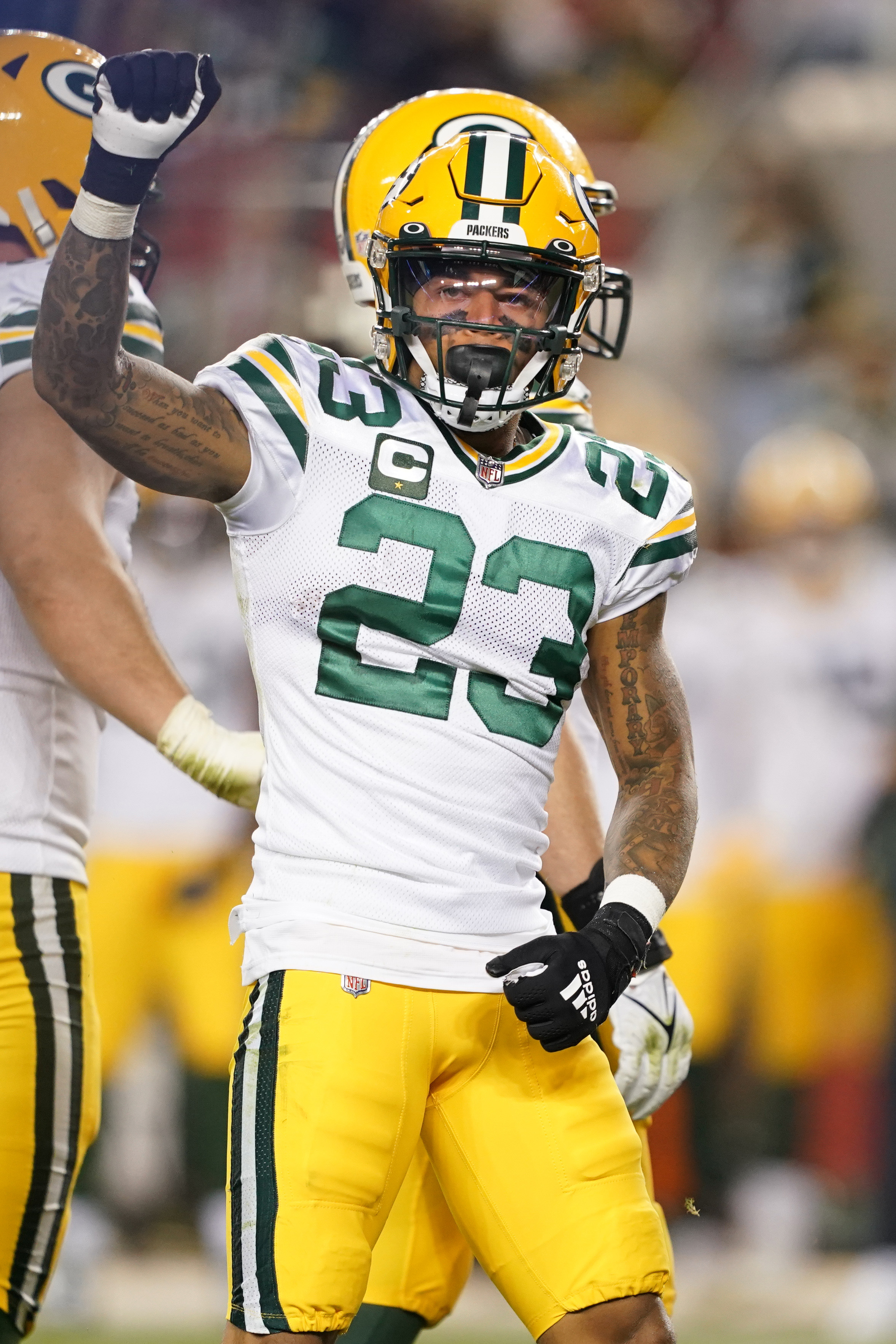A Green Bay Packers football player, wearing number 23, is celebrating during a game. He has his left arm raised in a fist near his yellow helmet which features a distinct white and green stripe. His white jersey, marked with the green number 23 and a captain's "C" insignia on his right shoulder, contrasts with his yellow pants that have a green and white stripe. He wears black Adidas gloves, a mouth guard, and has face paint on. The blurred stadium background shows other Packers players in similar attire—yellow helmets, white jerseys, and yellow pants, with one player partially visible to the left and another just behind him. The scene is brightly lit, indicating an outdoor, daytime game.